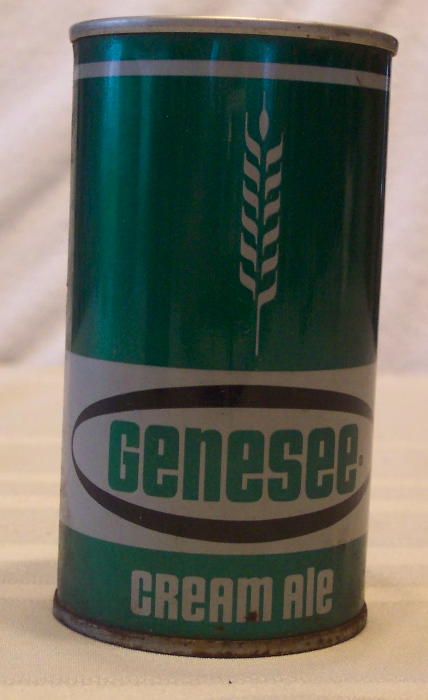This is a detailed photograph of a vintage-style beer can featuring a color palette of green, white, and black. The can shows signs of age, particularly noticeable on the rusted silver bottom area. The design is characterized by distinct horizontal stripes. At the top, there is a prominent green stripe adorned with a white wheat design. Directly beneath this, a white stripe displays the name "GENESEE" in bold letters, encircled by a black ring. Below this, a narrower green stripe bears the inscription "Cream Ale" in white lettering. The can is set against a plain white background, possibly a sheet, which accentuates its retro aesthetic and weathered condition.